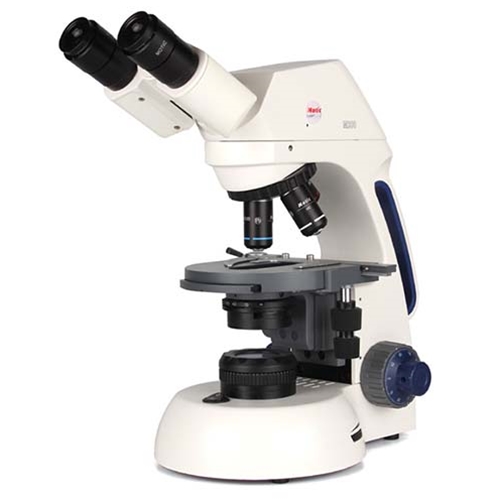This image features a sophisticated microscope showcasing a sleek design in black and white. The instrument is equipped with dual black eyepieces, ensuring comfortable and precise observation. A black focus knob is conveniently located at the bottom right for fine-tuning clarity. Beneath the stage, there's a light source that illuminates the specimens for better visibility. The revolving nosepiece at the top center holds three objective lenses of varying magnifications, allowing for versatile viewing options. The stage includes a secure tray with clips to firmly hold the slides in place during examination. The manufacturer's logo is prominently displayed on the right side, adding a touch of professional branding. Additionally, a power switch is situated at the bottom right for easy access to turn the microscope on and off.